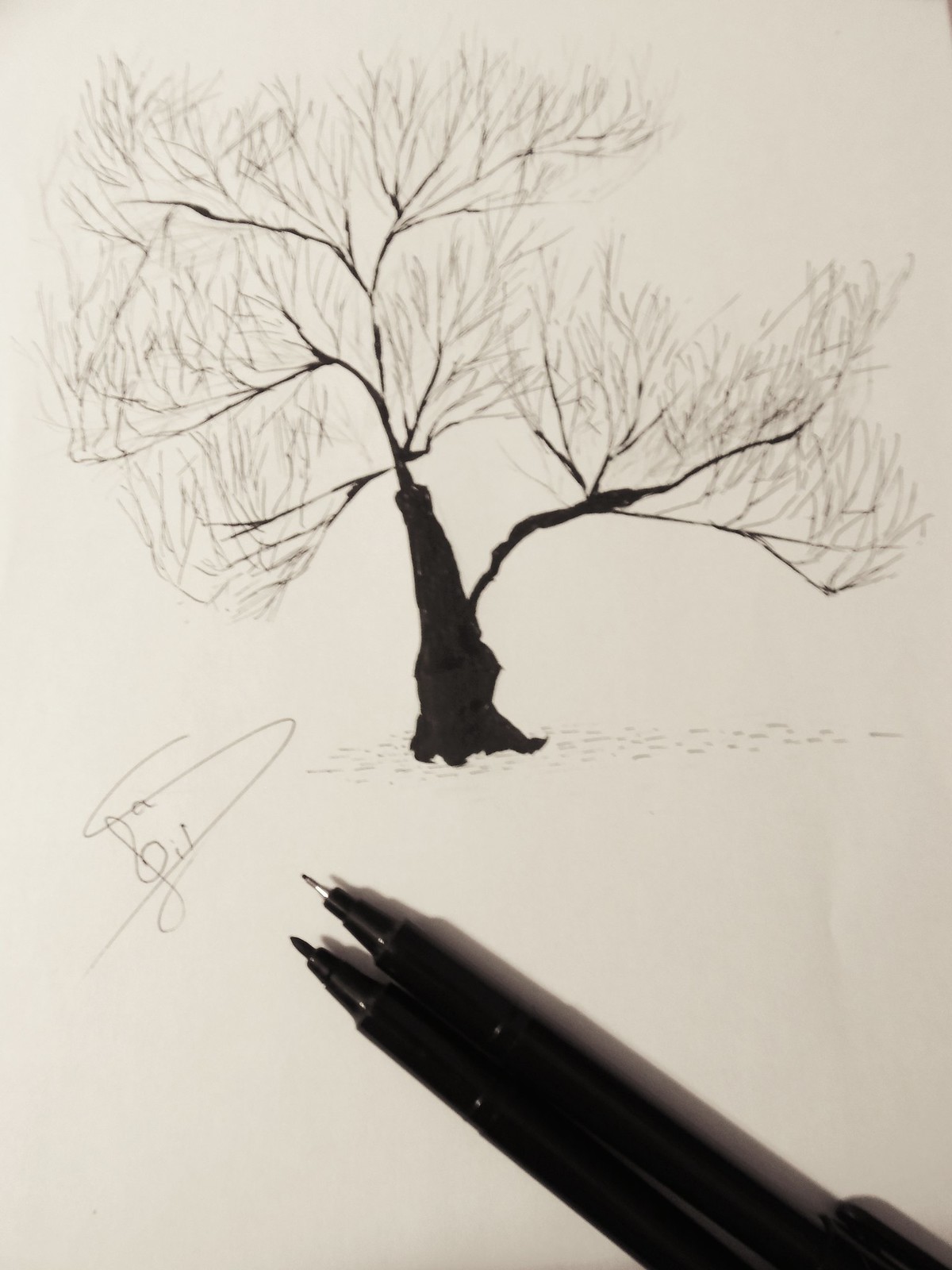This detailed pen and marker artwork, showcased on pristine white paper, captures a striking black tree with stark, branchless limbs stretching upwards. Positioned diagonally from the bottom right corner, the drawing instruments—a black pen and a black marker, both uncapped—serve as a testament to the artist's process. Near the base of the tree, subtle imprints on the ground evoke a sense of mystery, suggesting either footprints or fallen leaves. To the left of this intriguing scene, an elegant signature, resembling "Gill" in a sophisticated, stylized font, further personalizes the piece.